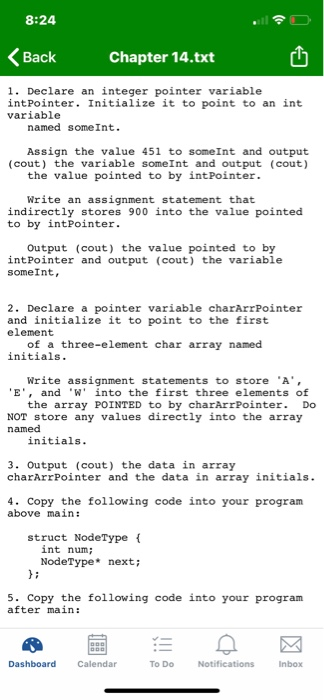In this screenshot of a home cell phone screen, the current time displayed at the top left is 8:24. On the top right-hand side, there are icons for signal strength, Wi-Fi connectivity, and battery life, which shows less than 20% remaining. Directly below this, in the center, the filename "chapter 14.txt" is prominently displayed. To the left of this title, there is a back arrow button, while a download icon is situated to the right.

Beneath the title, a series of numbered text sections are laid out in a vertical list format. The numbers are aligned to the left and range from one to five. Section one contains four sentences, section two includes two sentences, section three has one sentence, section four features one sentence along with some additional words below it, and section five comprises one sentence.

At the bottom of the screen, there are five icons arranged from left to right, labeled as follows: Dashboard, Calendar, To-Do, Notifications, and Inbox. Centrally located at the very bottom of the screen is a black horizontal bar.